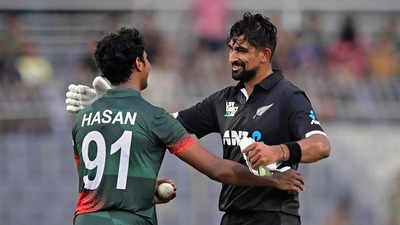In this landscape-style, colorized photograph, two male sports players of apparent South Asian descent—likely from India, Pakistan, or Bangladesh—are captured moments before embracing after a match. The player on the left, with his back turned to the camera, is wearing a green jersey with "Hassan 91" emblazoned on it and is holding a ball, possibly a cricket ball, in his hand. He does not have facial hair. The player on the right, facing the camera, is dressed in a black jersey adorned with some logo and writing. He is in his 30s, has a beard, and is partially gloved, holding one white glove in his hand while the other remains on. Both figures are sharply in focus against a blurred background suggestive of a cheering crowd, indicating a professional or semi-professional sports event, likely cricket, considering the attire and the ball.